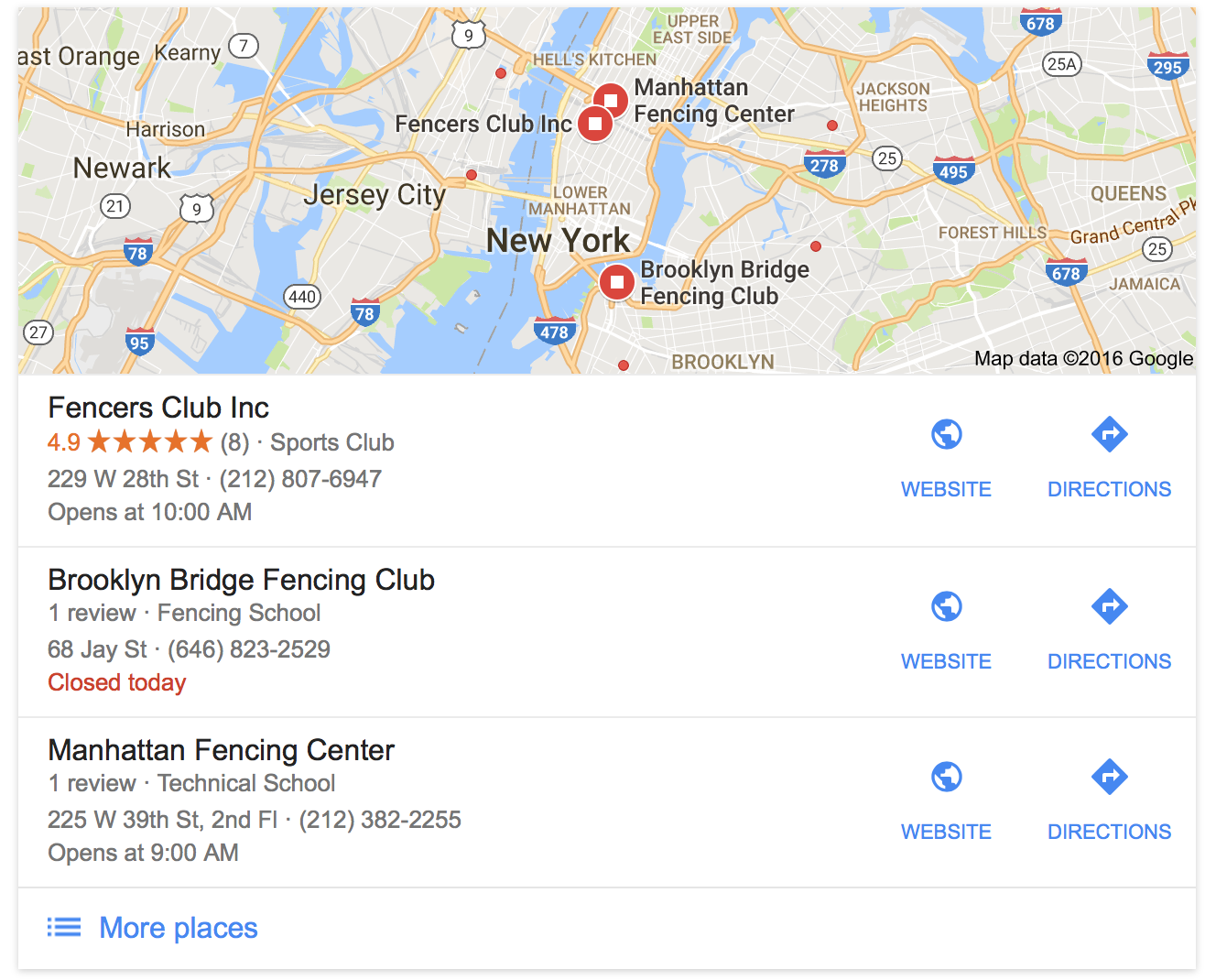**Detailed Caption:**

The image is a rectangular screenshot displaying fencing locations within New York City, slightly wider than it is tall to highlight its horizontal orientation. The map shows regions of New Jersey and New York, colored in muted gray tones with yellow interstates weaving through the area, while blue shades depict bodies of water.

Three distinct fencing clubs are marked on the map with red circles containing white squares. These include:

1. **Manhattan Fencing Center**:
   - **Location**: 225 West 39th Street, 2nd Floor, New York City
   - **Contact**: 212-382-2255
   - **Rating**: (One Review)
   - **Type**: Technical School
   - **Hours**: Opens at 9 a.m.
   
2. **Fencer's Club, Inc.**:
   - **Location**: 229 West 28th Street, New York City
   - **Contact**: 212-807-6947
   - **Rating**: 4.9 stars
   - **Type**: Sports Club
   - **Hours**: Opens at 10 a.m.
   
3. **Brooklyn Bridge Fencing Club**:
   - **Location**: 68 J Street, Brooklyn
   - **Contact**: 646-823-2529
   - **Rating**: (One Review)
   - **Type**: Fencing School
   - **Hours**: Closed today

Underneath the map, additional information for each fencing club is provided, ensuring a comprehensive understanding of their locations, contact details, ratings, and operational hours.